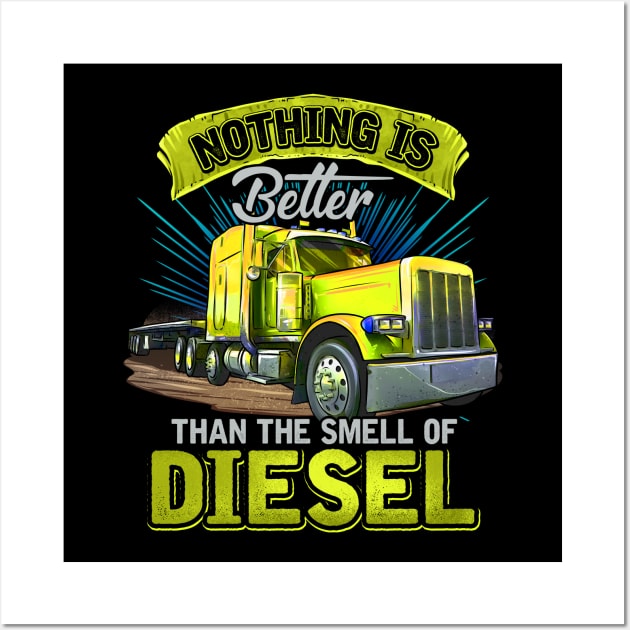This graphic design image depicts a large yellow tractor-trailer or 18-wheeler truck with a chrome grill, steel wheels featuring holes around the rims, prominent lug nuts, and a steel sidestep. It also has chrome mirrors extending from at least the passenger side. The truck is depicted with a flatbed trailer on a brown dirt mound. The entire scene is set within a black rectangle framed by a white border, creating a poster or banner-like effect.

The truck, with its big square hood and what appears to be a tinted yellow window, is accented by blue rays emanating from its rear, adding a dynamic element to the design. Above the truck, a ribbon-style label reads "Nothing is" in black letters on a yellow background. Below the truck, the words "better" and "than the smell of" are rendered in white and gray text, respectively, with "diesel" in prominent yellow letters.

The text layout in a masculine, all-capital font, emphasizes the sentiment: "Nothing is better than the smell of diesel," set against varying backgrounds of rusted green and gray, aligning both the strong industrial theme and the gritty aesthetic of the truck itself.